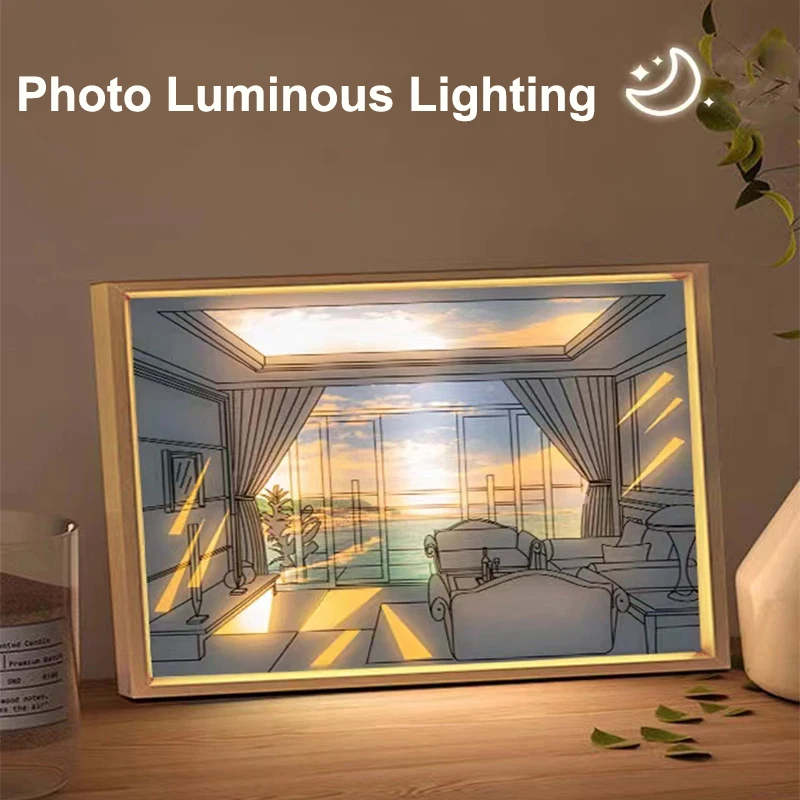The image showcases an advertisement against a brownish-beige wall, with bold white text at the top reading "Photo Luminous Lighting," accompanied by a small, clip-art style crescent moon and starburst symbols. Central to the image is a brown-framed illustration, leaning against the wall on a wooden table. The artwork within the frame is a detailed, hand-drawn sketch in thin black lines on a gray background, depicting an apartment interior with sofas, chairs, and tables. The room contains a prominent sliding door or large window with curtains, through which a vibrant seascape in color is visible, featuring an ocean and distant horizon at sunset. On the table, to the left of the frame, stands a scientific beaker filled with liquid, and to the right, there are dried leaves and the edge of a vase, with some flowers still attached to the stems peeking into the frame.